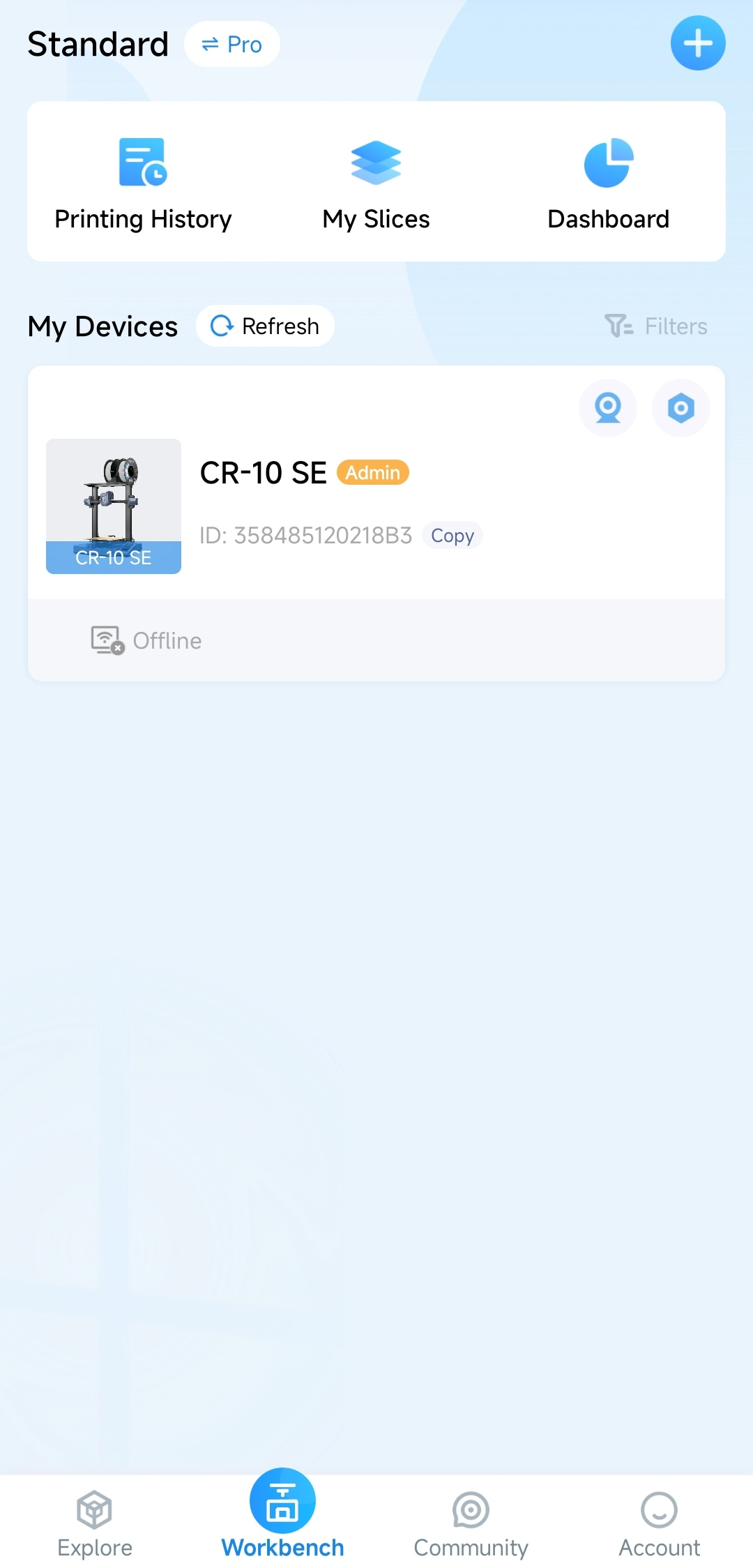In the image, the interface of a software application is displayed. At the top, there is a "Standard" label with a "Pro" button adjacent to it, indicating different tiers or versions of the software. Below this, there are main sections labeled "Printing History," "My Slices," and "Dashboard," indicative of key functionalities offered by the application. At the bottom of the interface, additional tabs labeled "Explore," "Workbench," "Community," and "Account" provide further navigation options. The current view is focused on the "Workbench" section.

Within the "Workbench," there are subsections including "My Devices." Here, there is an image of a tool bench-like structure. This structure appears to be a stool-like table with spools on top, and a ring-like arrangement around the legs, possibly for support or aesthetic purposes. The device in focus is identified with a label "CR-10SE," and the user is listed as an "Admin," indicating ownership or control over this device. Additionally, an ID beginning with "358" is visible, likely serving as a unique identifier for the device within the application. This detailed view suggests a workspace where the user can manage and control various devices associated with their account.